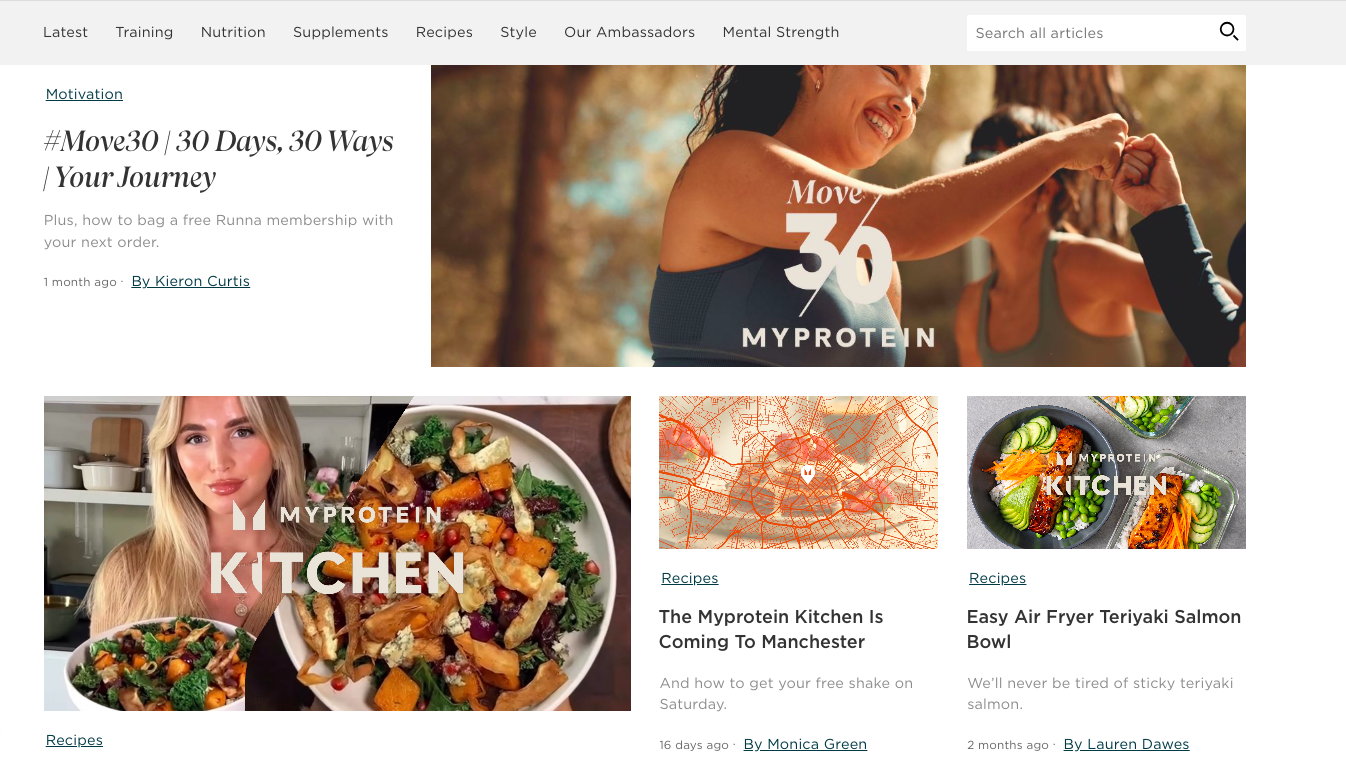Here is a revised and detailed caption for the image:

---
This screenshot captures a portion of the MyProtein website, specifically highlighting the layout and elements found on one of their webpages. At the top of the page, a gray navigation banner is prominently displayed. It includes various categories: "Latest," "Training," "Nutrition," "Supplements," "Recipes," "Style," "Our Ambassadors," and "Mental Strength." Adjacent to these categories, on the right side, is a search bar featuring the placeholder text "Search All Articles."

Below the navigation banner, the main content area of the webpage has a clean, white background. In the top left corner, a small blue hyperlink labeled "Motivation" is visible. Beneath this link, a bold header reads, "Hashtag Move 30, 30 Days, 30 Ways, Your Journey," along with a subheader that advertises, "Plus, How to Bag a Free RUNA Membership with Your Next Order." This is followed by a timestamp marked "Posted one month ago" and a hyperlinked author name.

To the right of this text, there is a large horizontal rectangle featuring a photo background. The image depicts a woman giving another woman a fist bump, overlayed with the text "Move 30, MyProtein" at the bottom.

Further down the webpage, thumbnail previews of various articles are displayed. These include sections like "Recipes" and additional articles, offering a glimpse into the diverse content available on the website.
---

This caption not only organizes the information more clearly but also provides a detailed and comprehensive description of the webpage's layout and content.